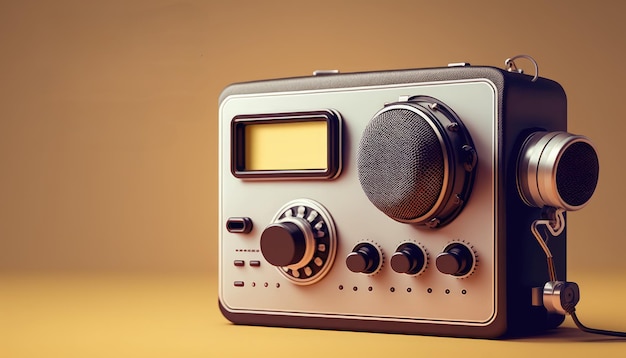The image features a detailed close-up of a modern, stylized radio device, positioned on a yellowish platform against a gold-toned background that darkens towards the upper section. The radio, which occupies the right side of the photograph, has a silver faceplate encased in a black frame. Prominently, it showcases a series of four black knobs: three smaller ones aligned horizontally, plus a larger knob situated adjacent to the smaller ones. There is a notable round speaker grille on the right-hand side of the face, resembling a microphone grill. 

The centerpiece of the radio is a rectangular LED screen with a yellow tinge and a black border, currently turned off. Below this screen, additional buttons are visible, along with some indistinct writing at the bottom of the device. Noteworthy details include a peg on the right side, possibly for attaching a strap, and a connector with a wire emerging from the lower section, extending to the right. Overall, the radio exudes a high-quality, premium design, though it lacks any discernible branding or labels.